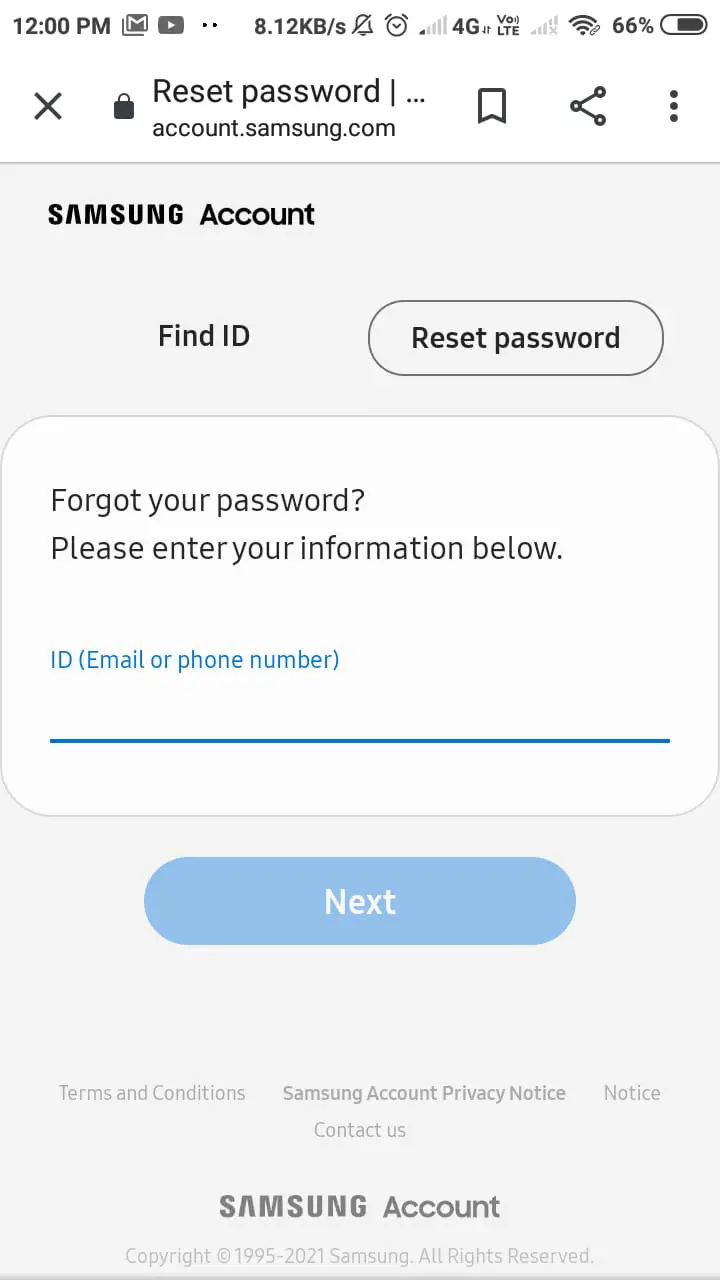An image displayed on a smartphone screen shows a detailed view of the Samsung account password reset page. The phone's status bar at the top indicates a battery life of 66%, a strong 4G connection with only one bar, and the time as 12:00 PM. The webpage is accessed via the URL "account.samsung.com," and features a lock icon and an 'X' on the left, and a box-like icon on the right. 

The page is divided into sections with a clean, gray background. Prominently, "SAMSUNG ACCOUNT" is written in all capital letters, followed by a "Find ID" link and a "Reset password" button with rounded edges. In the center of the page, a white box prompts users with "Forgot your password? Please enter your information below." Below this prompt are the fields for "ID, Email or Phone Number," highlighted in blue, followed by a faint blue "Next" button with white text.

Towards the bottom, the page lists additional options and notices in smaller text, including "Terms and Conditions," "Samsung Account Privacy Notice," "Contact Us," and another instance of "Samsung Account" at the very bottom.